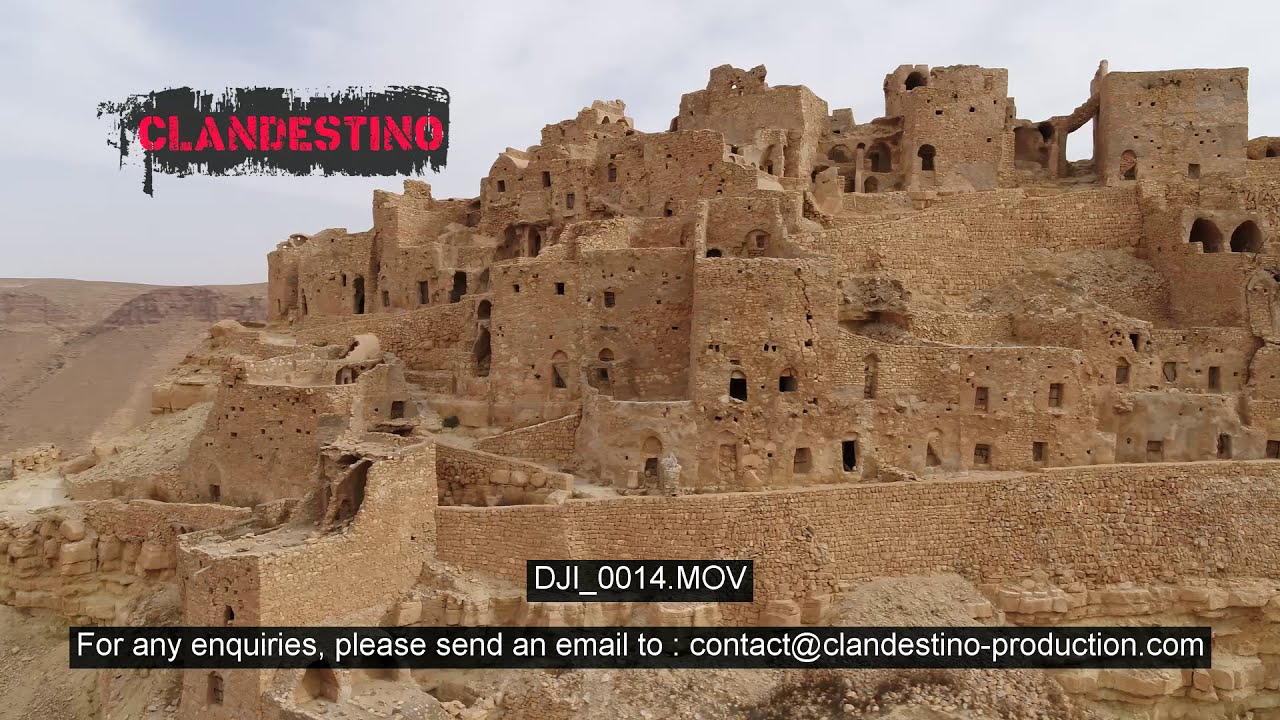The image depicts a troglodyte village carved into a mountainside, likely situated in the Middle East, Albania, or Tunisia. The ancient city, constructed from rusty tan sandstone, is characterized by its multi-level, cave-like structures, some of which are decayed and open to the elements. In the foreground, there is a large stone wall. The scene is framed by visual elements suggestive of a promotional screenshot: in the top left corner, a black, paint-stroke-like background with red capital letters spells out "CLANDESTINO." Below this, small black boxes contain white text, including "DJI_0014.MOV" and a contact email: "contact@clandestino-production.com."